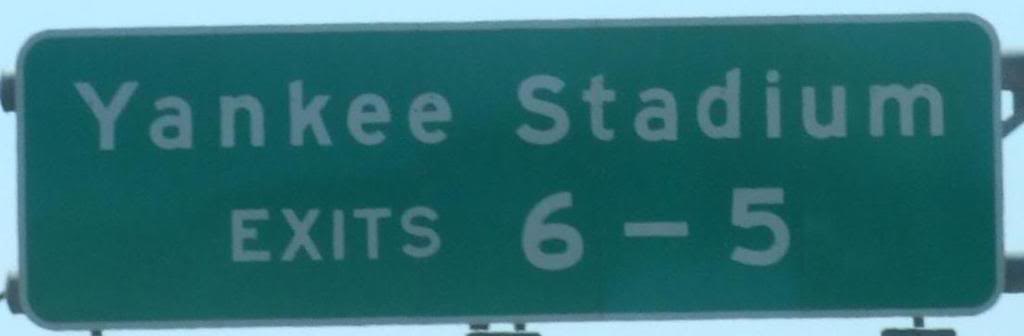A green street sign directing motorists to Yankee Stadium exits 6 and 5 dominates the image. The text on the sign appears gray in the photograph, but it is presumably white. The sign is set against a clear blue sky, suggesting a bright, sunny day. The photo is closely cropped, focusing solely on the street sign itself, with the edges of the metal mounting pillars just barely visible. There are no other objects in the frame, emphasizing the importance of the sign's directions to Yankee Stadium.